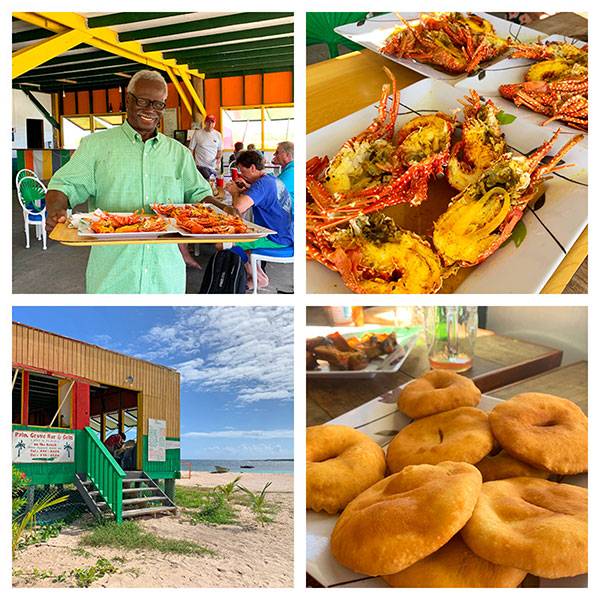The composite image is divided into four smaller square images arranged in a grid. In the top left corner, there is a dark-skinned man with gray hair, wearing black glasses and a mint green collared shirt. He's holding a yellow tray with three white square plates filled with various seafood, possibly lobster, crabs, and prawns. Behind him, there's a colorful restaurant interior with an orange wall, green ceiling slats, and a white accent. People are seated at tables in the background, enjoying their meals. The top right image is a close-up of the seafood on the plates, revealing detailed, prepared crabs with white plates that have decorative stems and stalks drawn on them. The bottom left image shows the exterior of the restaurant: a one-story shack located beachfront, made of tan and green slats with a green bannister leading up a stairway. The sky above is blue with white clouds and there’s a sandy beach surrounding the shack. Lastly, the bottom right image features a wooden table with a glass containing very little liquid and a plate of golden brown donuts or muffin-like desserts.